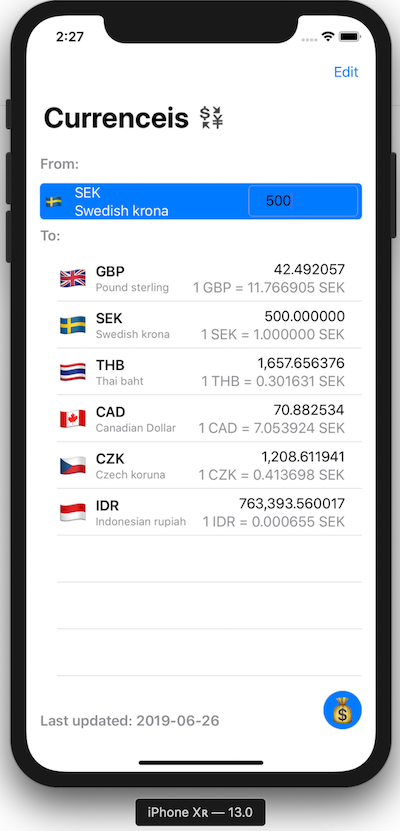Screenshot of an iPhone XR13 displaying a currency conversion application. The top information bar indicates the current time as 2:27, shows a full battery charge, and a strong internet connection. In the app, "Currencies" is misspelled as "C-U-R-R-E-N-C-E-I-S". The interface lists various currencies with "SEK" (Swedish Krona) highlighted, suggesting the user may be located in Sweden. The conversion rates shown are as follows:

- SEK 500 to:
  - GBP (British Pound Sterling): 42.49
  - THB (Thai Baht): 1,657.656
  - CAD (Canadian Dollar): 70.882
  - CZK (Czech Koruna): 1,208.61
  - IDR (Indonesian Rupiah): 763,393.560

This information was last updated on 2019-06-26. The user appears to be checking the value of 500 Swedish Krona in various other currencies.